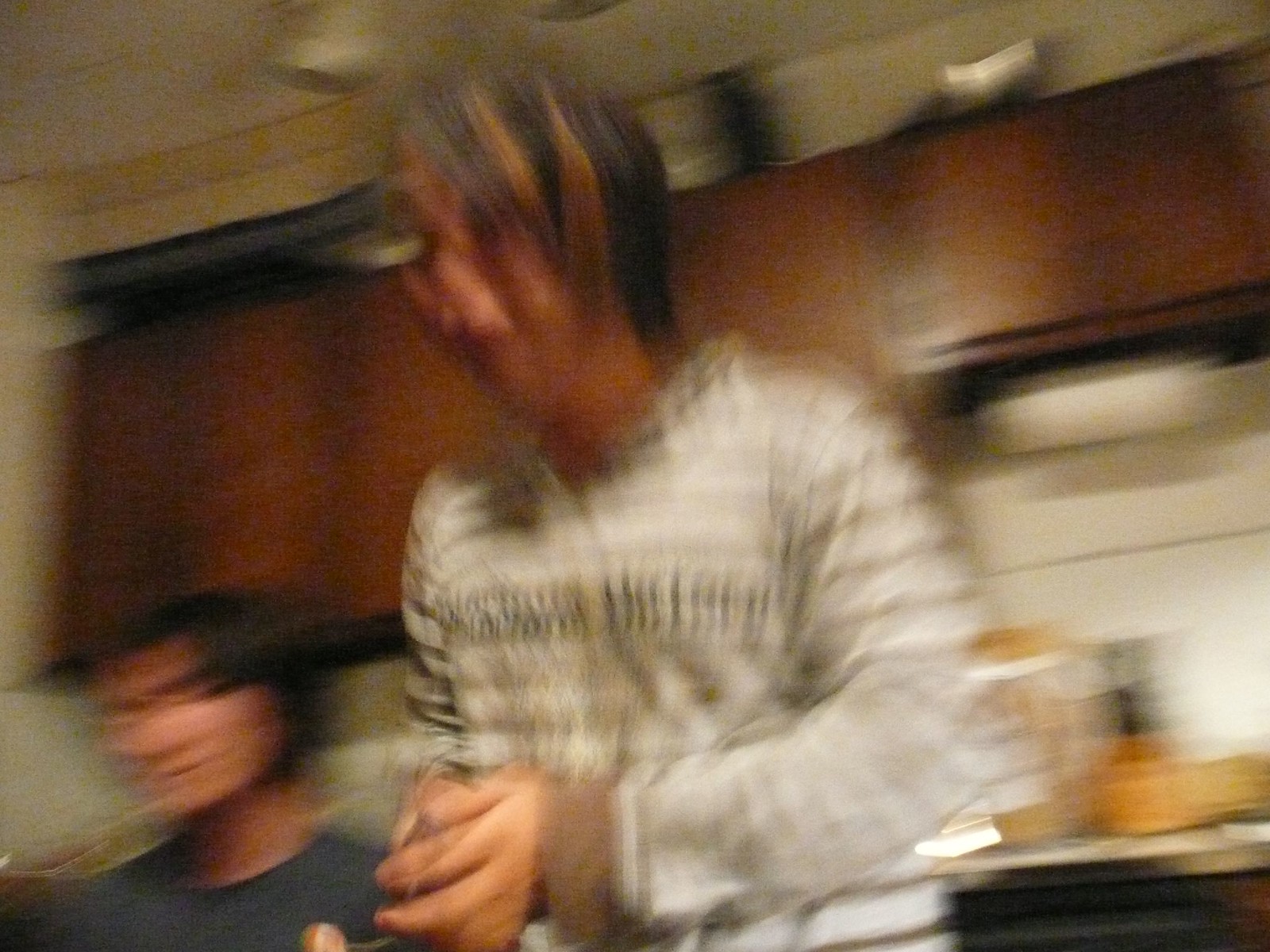The photograph is a very blurry indoor shot taken inside a kitchen. The camera is angled diagonally upwards towards the top left, capturing a segment of the kitchen's upper cabinets which are dark brown in color. Below the cabinets, a white wall is partially visible, along with a small portion of a countertop that appears to be either white, light gray, or silver. Some indistinct brown items rest on the countertop. In the bottom left corner, a male figure with light skin, black hair, and wearing a gray shirt is visible. In the center of the image stands another individual with medium-colored skin and black hair streaked with lighter shades. They are wearing a long-sleeved white t-shirt adorned with horizontal stripes and have their hands clasped in front of them.